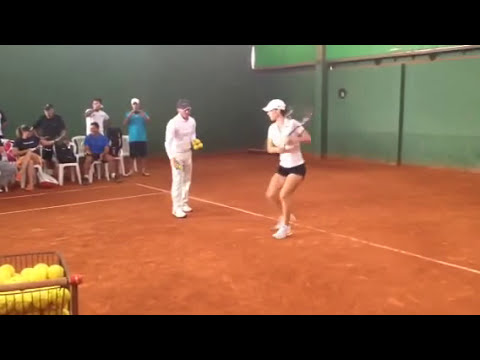The photo captures the interior of a gymnasium or tennis court with a brown clay floor. In the lower left-hand corner, there is a black mesh basket full of green tennis balls. At the center of the image stands a woman engaged in tennis practice, poised to hit a backhand. She is dressed in a white baseball cap, a white t-shirt, black shorts, and white sneakers, and holds a tennis racket. Opposite her, an older man in white attire—white shirt, white pants, white sneakers, and a gray cap—holds several tennis balls in one hand and is about to toss one with the other.

The background features a green wall and a group of five people seated on white plastic chairs. Among them, a man in a blue shirt with a white hat converses with a woman wearing a black shirt. Another man in a black shirt and black cap, a man in a white shirt, and a man in a blue shirt observe the scene. One person appears to be taking pictures. Black framing is visible at the top and bottom of the photo. Several people behind the trainer seem to be watching the practice session, and the court is marked with standard tennis lines.